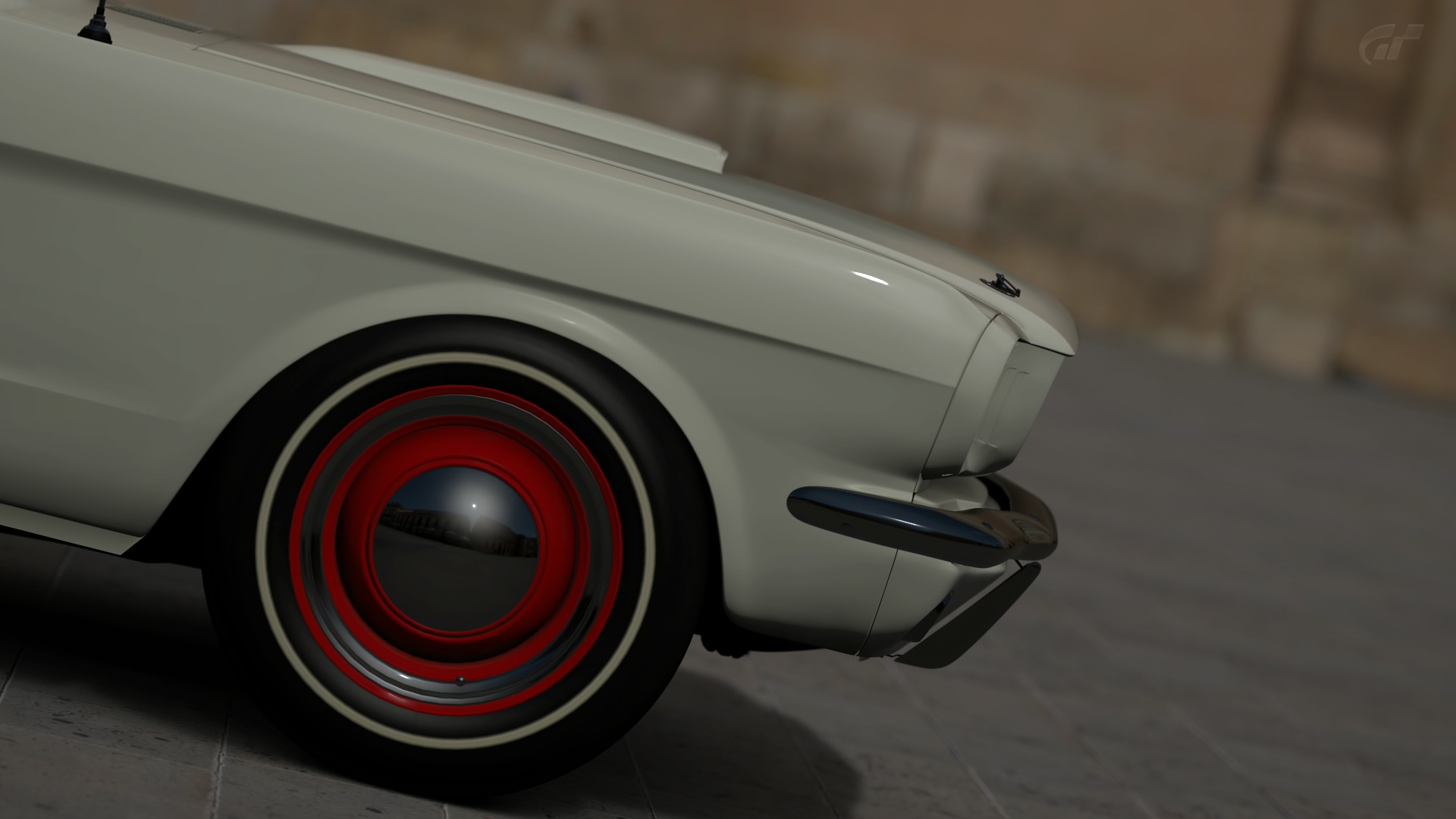The image depicts a close-up view of the front end of a sleek, exceptionally low-profile car with a highly reflective, pristine white finish. The focal point is an intricately designed tire featuring a striking color transition: it starts with a black outer tread, followed by a whitewall, then a bold red stripe, a gray band, another red section, and finally a shiny gray hubcap. The car's bodyline emerges from the center and upper left of the image, extending towards the lower and middle right. In the background to the right, a vague, gray surface suggests the car is parked on a neutral ground, while the upper and central portions of the right background reveal an indistinct, out-of-focus brown stone area, adding a hint of environment to the scene.